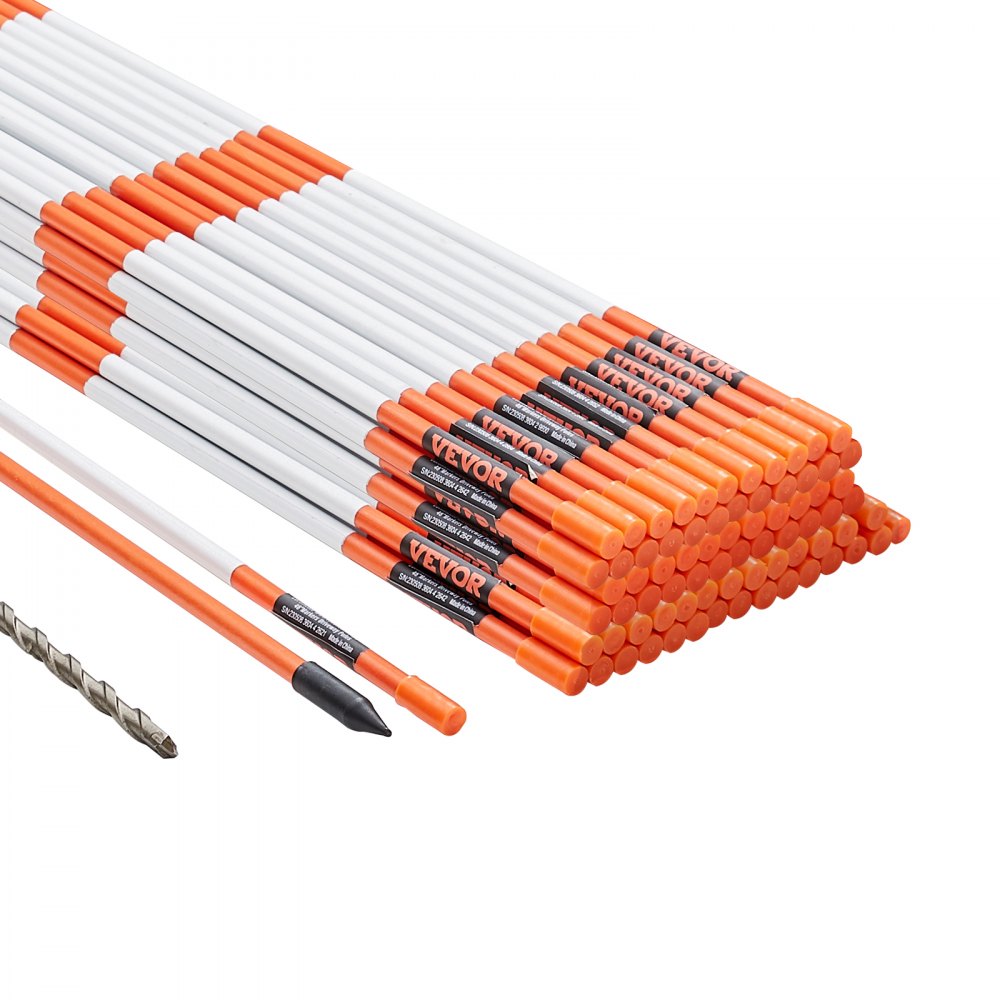The image depicts a large stack, likely four or five dozen, of long, white, pencil-shaped objects with orange accents. These objects are not made of wood; rather, they appear to be plastic or some other non-wood material. Each unit is capped with an orange end and features an orange stripe around the middle and the bottom, the latter displaying the brand name "VIVOR." The items start in the top left corner and span diagonally to the bottom right of the frame, extending out of the picture at the top. Among the mostly uniform white-and-orange objects, there is one distinctive white stake with an orange cap and label, positioned next to a completely orange object that appears to have a pointed tip, possibly an electronic stylus. Additionally, a long, silver metal drill bit is seen in the bottom left corner. The background of the image is plain and white, providing no other context or details.